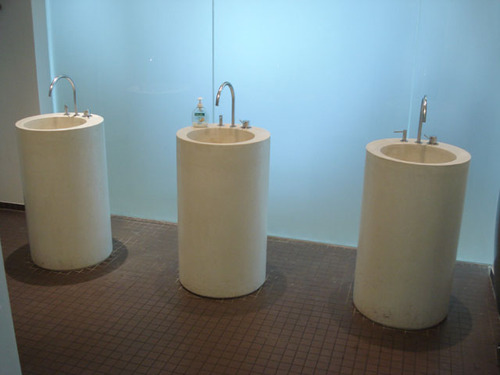The image depicts a realistic, horizontally-oriented photograph of what appears to be a public bathroom. The floor is covered in 4-inch by 4-inch brown ceramic tiles with dark grout lines. The background features a light blue, milky, backlit glass panel that adds a decorative touch, though it is not transparent. On the left side of the image, there is a partial white wall divider. 

Centered in the image are three modern, standalone cylindrical sinks. These sinks are white, possibly made of stone or hard plastic, and are arranged in a row spaced about two to three feet apart. Each sink has a top cut out like a bowl to allow for water to collect, with a stainless steel, hooked-shaped bathroom faucet and two handles attached. The middle sink has a hand soap bottle situated on its surface, while the other two sinks do not have soap. The overall scene is well-lit and exudes a contemporary and clean atmosphere.